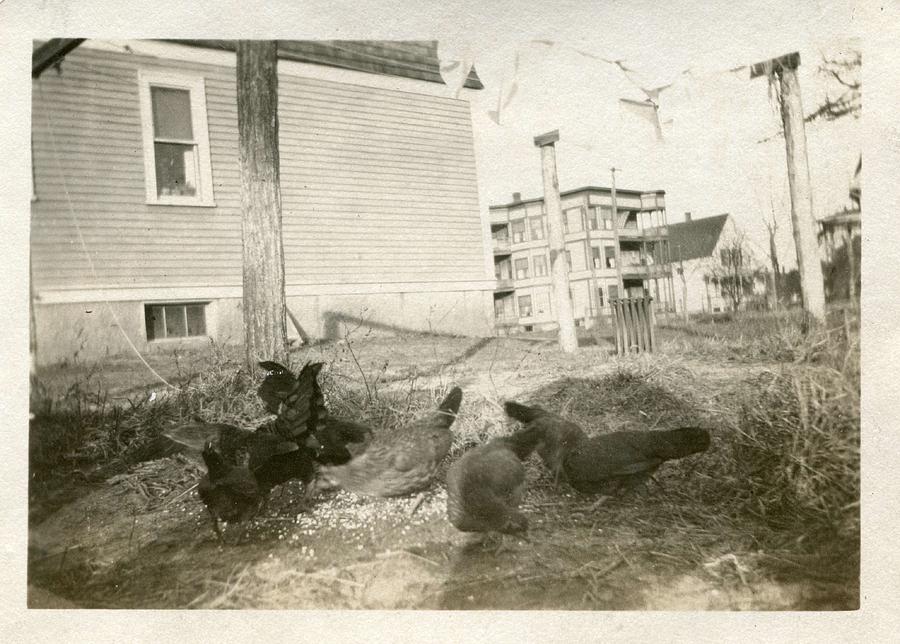The image is an antique black-and-white photograph taken in a residential area, capturing a moment in time that feels both historic and somewhat eerie. At first glance, the photo is grainy and hard to decipher, requiring a closer look to appreciate its details. In the foreground, there are several chickens—seven by count—pecking at the ground, which is a patch of dirt interspersed with dry sticks and some tumbleweed. The birds appear to be in motion, their heads down, likely pecking at some feed.

Moving to the mid-ground, a clothesline strung between poles stretches across the scene, draped with white clothes, adding to the nostalgic ambiance. The background is dominated by two buildings: one that looks like a typical house with shattered glass, hinting at either age or damage from thrown rocks, and another structure that is larger and could either be a substantial house or an apartment building. These buildings are run-down and shabby, with tall, dead grass and weeds surrounding them, reinforcing the photograph's old and desolate atmosphere. The entire scene is devoid of color, enveloped in shades of white, gray, and black, which further emphasizes the photograph's age and the lifeless state of the environment.